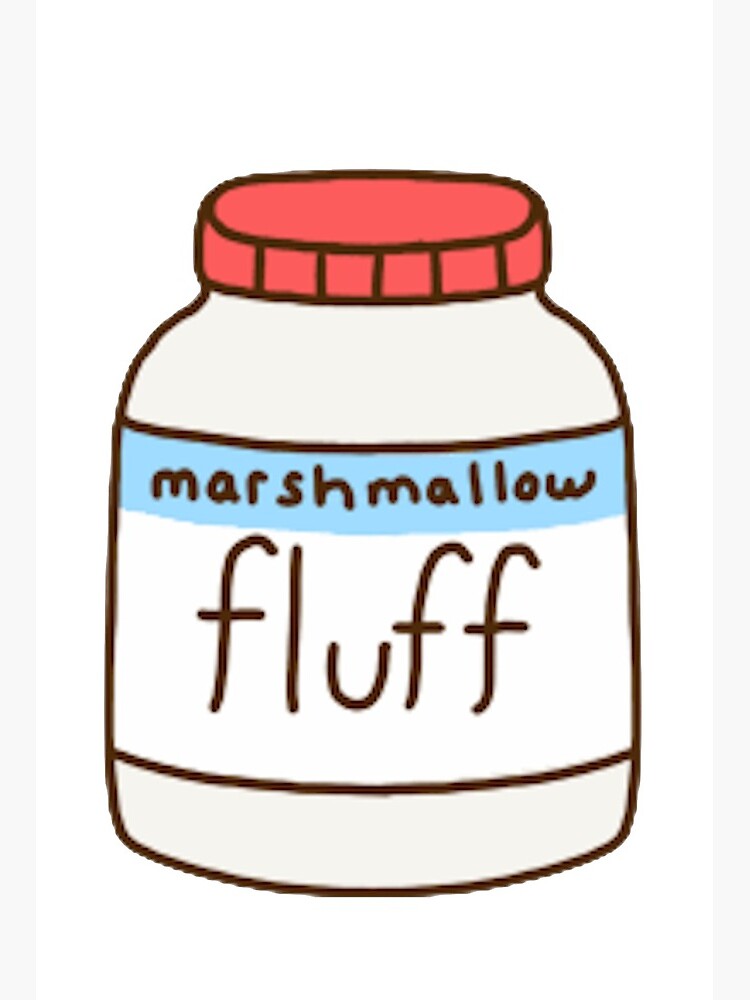This image is a cartoon drawing set against a white background with darker white bands framing it on the left and right. At the center of the image is a large, white jar with a black outline. The jar has a rounded, vertical shape and is topped with a red cap that features small, vertical black lines. The front of the jar is adorned with a label that is mostly white. The upper portion, approximately one-fifth of the label, is light blue and displays the word "marshmallow" in all lowercase black letters. Beneath this, taking up the majority of the label, the word "fluff" is written in larger, black lowercase letters. There is also a black stripe beneath the word "fluff." Overall, the label on the jar reads "marshmallow fluff." This hand-drawn illustration effectively depicts a container of Marshmallow Fluff.